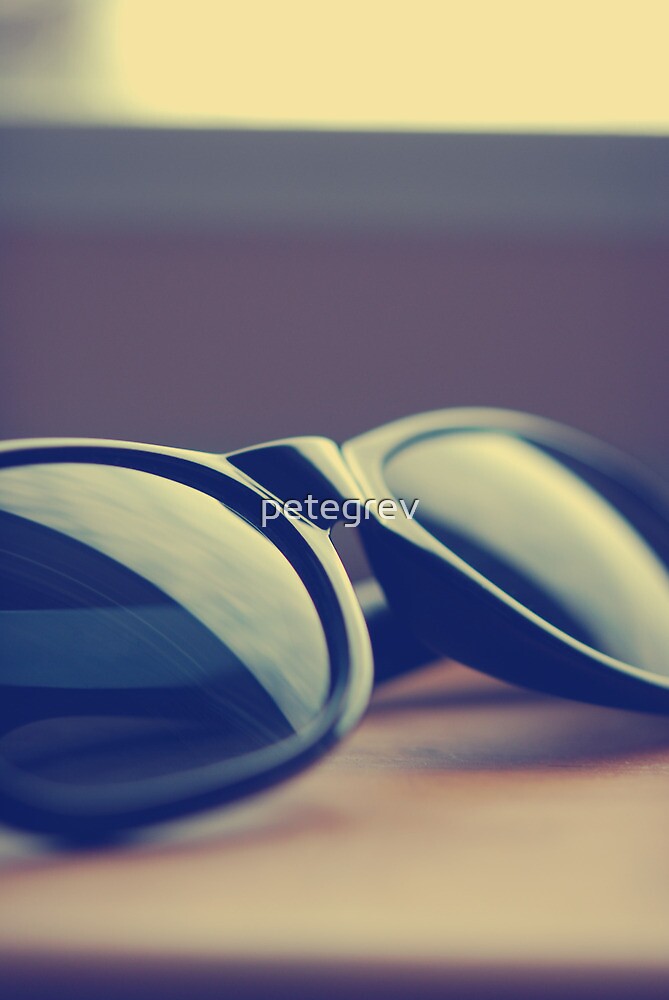A pair of folded sunglasses is the central focus of this image, resting on what appears to be a wooden table. The photograph features a blurred background, making it difficult to discern the setting, though it suggests an indoor environment such as a classroom or an office. The sunglasses, positioned towards the bottom-center of the image and angled upwards diagonally, have a simple design with black, glossy black, and tinted rims. The lenses and frames both appear dark, likely black. The colors in the image include various shades of brown from the table and a mix of white, off-white, gray, and black in the background. A watermark, reading "Pete Greve," is prominently displayed directly over the sunglasses, indicating either a brand or a watermark.